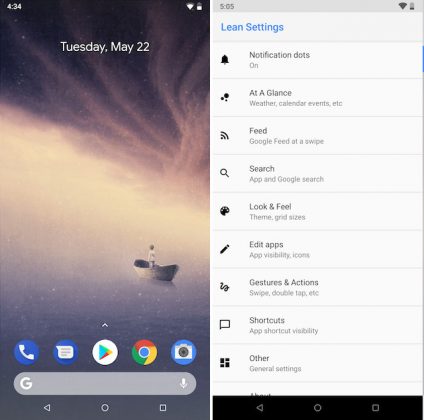This is a detailed caption for an image of a smartphone screen:

---

In the top-left corner of the smartphone screen, the current time is displayed in a white font as "4:34." Towards the top-right corner, icons for Wi-Fi and battery life are visible. The battery icon indicates a low charge. The background of the screen is dark gray, with the date "Tuesday, May 22" shown in white font near the center. 

The main background image features a scene of grayish clouds, with a person in a gray boat wearing white, floating on the water. 

Below the primary background image, a series of circular app icons is arranged horizontally:

1. A blue circle with a white phone icon.
2. A blue circle with a white document icon.
3. A white circle with a triangular logo in red, orange, and teal, resembling a Microsoft app.
4. The Google Chrome icon.
5. A blue circle with a white camera icon, featuring a gray internal design.

Beneath these icons, there is a gray elongated circle housing:

- The Google "G" logo on the left.
- A white microphone on the right.

At the bottom of the screen, there are navigation icons including:

- A white triangle pointing to the left.
- A white circle.
- A white square.

Towards the bottom-right, the time "5:05 p.m." is displayed once more in black text. Adjacent to this are icons for Wi-Fi and battery life again, with the battery icon still indicating a low charge. Below this, there is text on a white background with blue letters that reads "Lean Settings."

Further down, a series of options is displayed on a white background with black font and icons:

- A bell icon marked with notification dots, followed by "At a glance," including weather, calendar events, etc.
- A Wi-Fi icon labeled "Feed Google," followed by "Feed at a swipe."
- A magnifying glass icon labeled "Search app" and "Google search."
- A half-circle icon for "Look and feel theme," "Grid size."
- A pencil icon for "Edit apps," "App visibility," "Icons."
- A squiggly line for "Gestures and actions," including "Swipe," "Double tap," etc.
- A square icon for "Shortcuts," "App shortcut visibility."
- A series of small squares next to "Other general settings."

At the bottom, there is a black box with a gray outline containing:

- A triangle pointing to the left.
- A gray circle.
- A gray square.

---

This caption provides a comprehensive breakdown of the various elements visible on the smartphone screen.